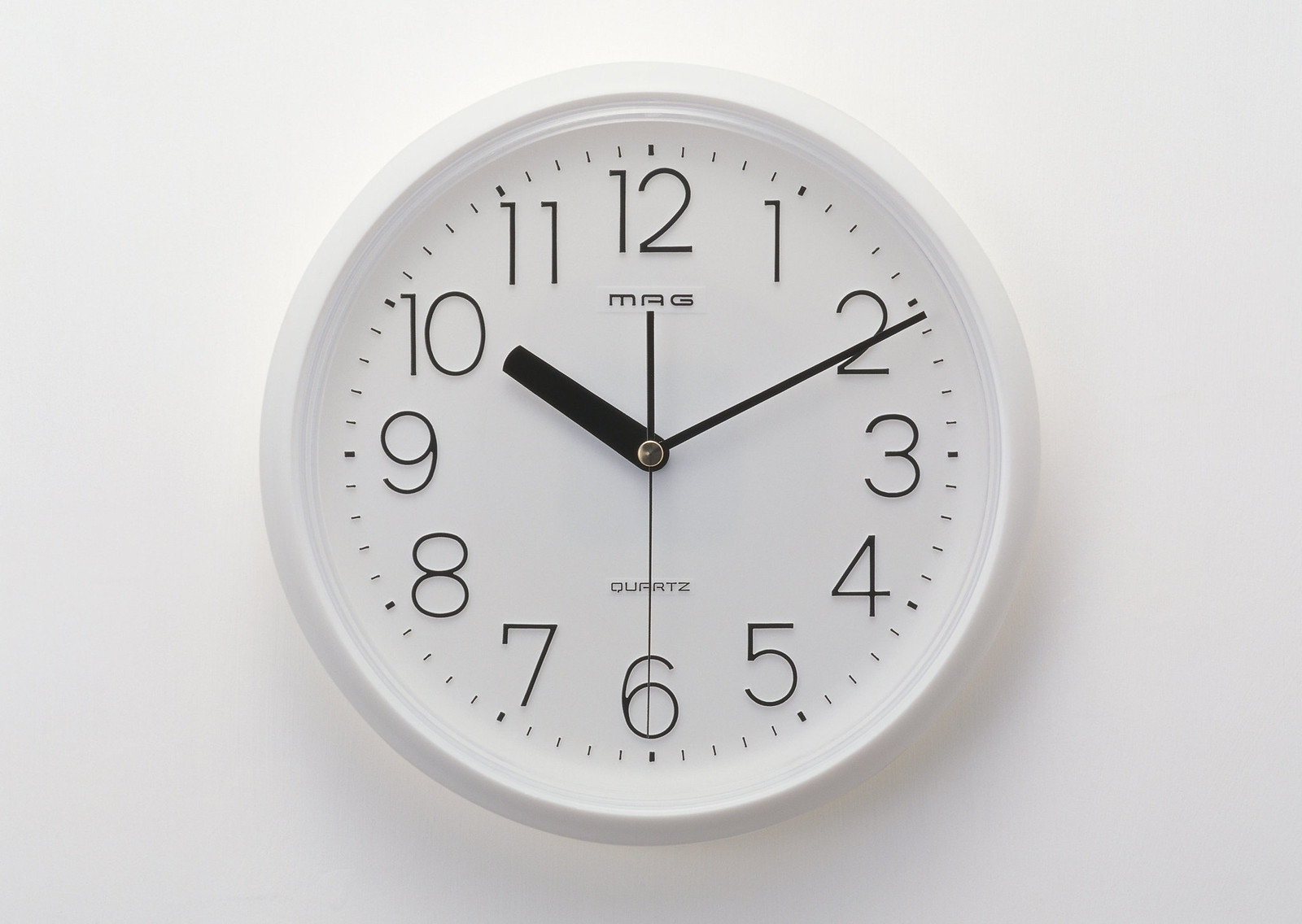This high-quality photograph features a centrally placed, round clock set against a solid white background. The clock, which takes up the majority of the image, has a white casing and a white face. Black numerals mark the hours, with thin lines delineating the minutes between them. The clock shows the time as 10:10 and 30 seconds; the hour and minute hands point to the 10 and 2 respectively, while the black second hand aligns with the 6. Just below the 12 o'clock position, the brand name "MAG" is inscribed, and above the 6 o'clock position, the word "quartz" is visible in small lettering. The clock hands are black, and the center where the hands connect shows a slightly tarnished, faded copper color, indicating a minor wear in contrast to the otherwise new appearance of the clock. A subtle shadow cast by the clock adds depth to the otherwise simple white background.